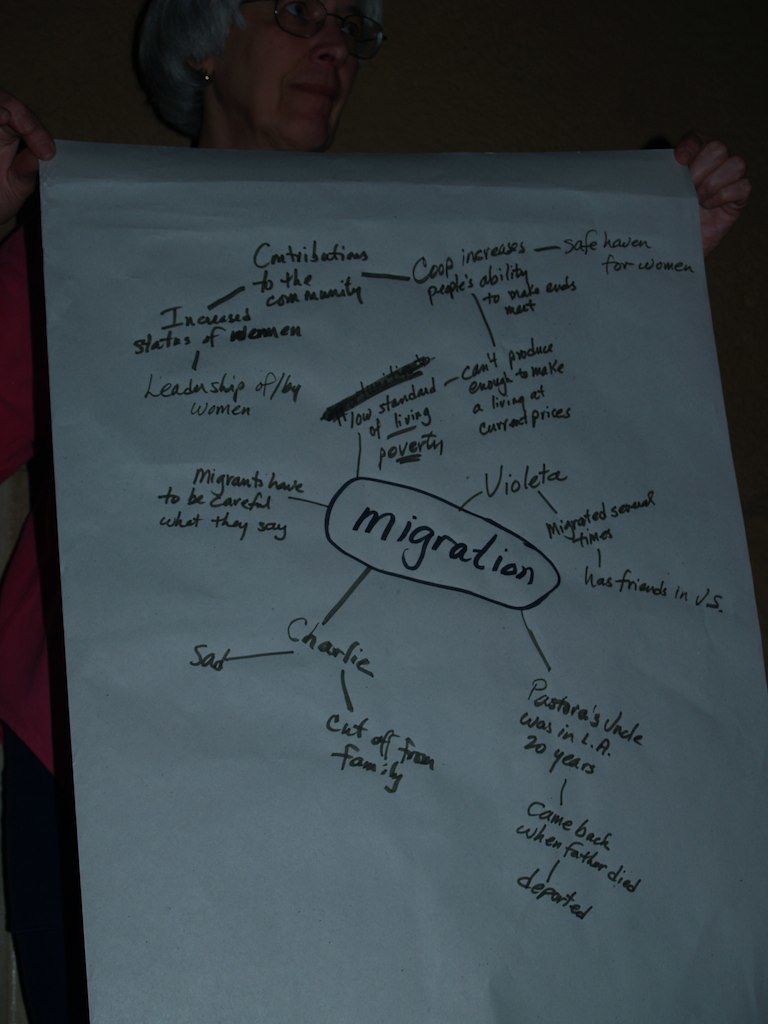In the foreground of a dimly lit setting, a woman holds a white paper sign covered in various handwritten notes. At the center of the paper, the word "migration" is prominently displayed within an elongated, uneven circle outlined in blue. Extending outward from the central word are multiple lines connecting to various names and details, forming a complex web of relationships and notes. 

Key names such as Violetta and Charlie are connected to phrases like "friends in JS," "sad," and "cut off from family." Notably, a separate line details that "Pastora's uncle was in LA 20 years, came back when father died," followed by "deported." Another area of the paper includes community-related notes in black ink, such as "contributions to the community," "increased state of," "leadership by women," and "safe haven for women." These notes are somewhat difficult to read due to poor lighting and irregular handwriting, obscuring some text. The document appears to be an intricate detailing of family connections, migration history, and community contributions, despite the challenges in legibility.